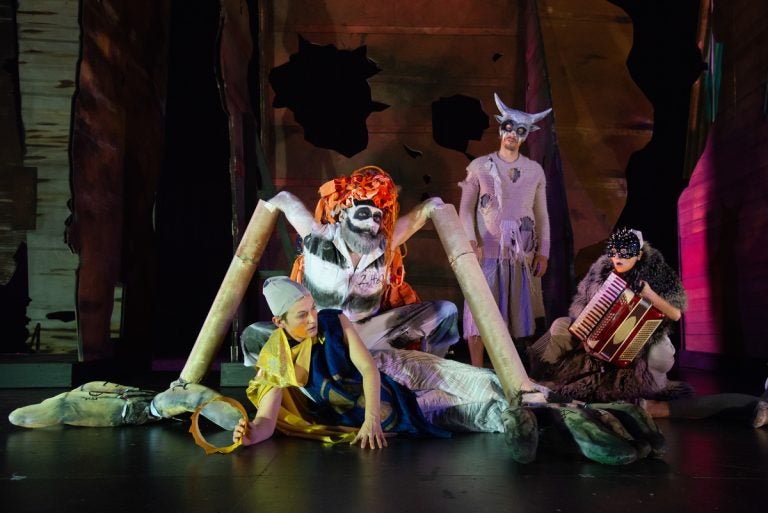This image depicts a stage set for a theatrical play or reenactment featuring four costumed characters. At the forefront, a young white woman lies on her side with a silver swim cap on her head, draped in blue and yellow fabric. She holds a tambourine, capturing a pivotal moment that exudes a sense of drama. Looming over her is a bizarre, spider-like figure with white face paint, a fake gray beard, and a flamboyant, bright red wig or headdress. His arms are replaced by elongated cardboard tubes, adding to his eerie, skeletal appearance reminiscent of Beetlejuice.

In the background, there are two more enigmatic characters. One wears a mask resembling a cow or demon, with silver horns, and a spotted dress, contributing to the surreal atmosphere. Next to this masked individual, a person with long black hair crouches, gripping an accordion. Their fur costume and intense, disconnected gazes amplify the scene's unsettling aura. The stage’s backdrop, featuring flat wooden or cardboard props and some red curtains, hints at a modest, possibly community theater production. This intricate tableau captures a moment rich with theatrical tension and eerie, fantastical elements.